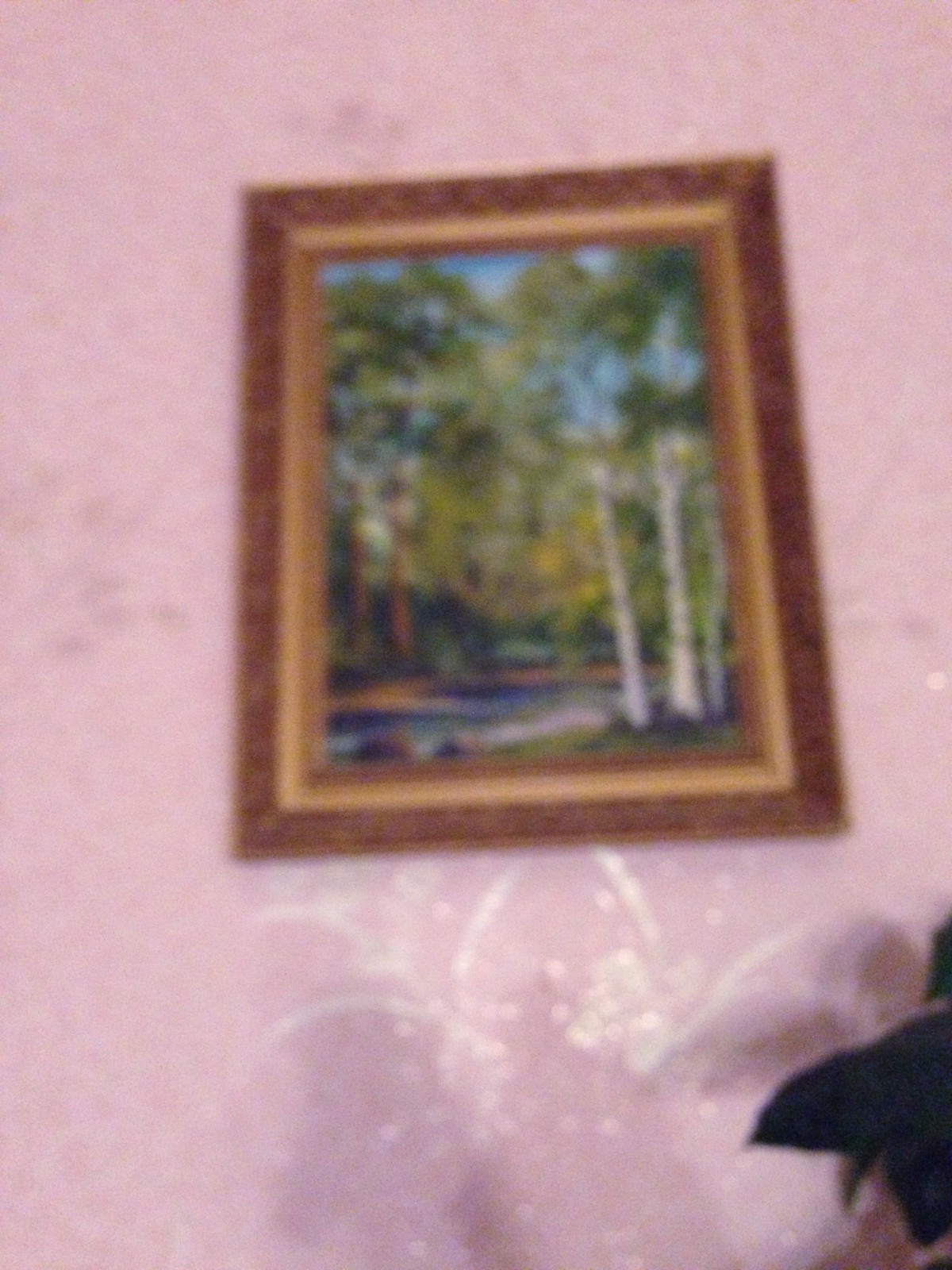This image features a very blurry photograph of a pink wall adorned with white, scratch-like marks. At its center, a large painting is prominently displayed in an ornate wooden frame that features golden trim. The artwork depicts a vibrant natural scene dominated by tall, slender trees. On the right side, two trees with distinctive white bark and green, billowing leaves stretch towards a bright blue sky, likely birch trees. On the left side, the trees have brown bark with similar green foliage. Below this arboreal display, hints of a water body are visible, winding through a grassy and possibly dirt-strewn landscape. In the background, there are more diffuse elements, possibly representing bushes and a blurred sunset, casting a yellowish light that blends into the scene.